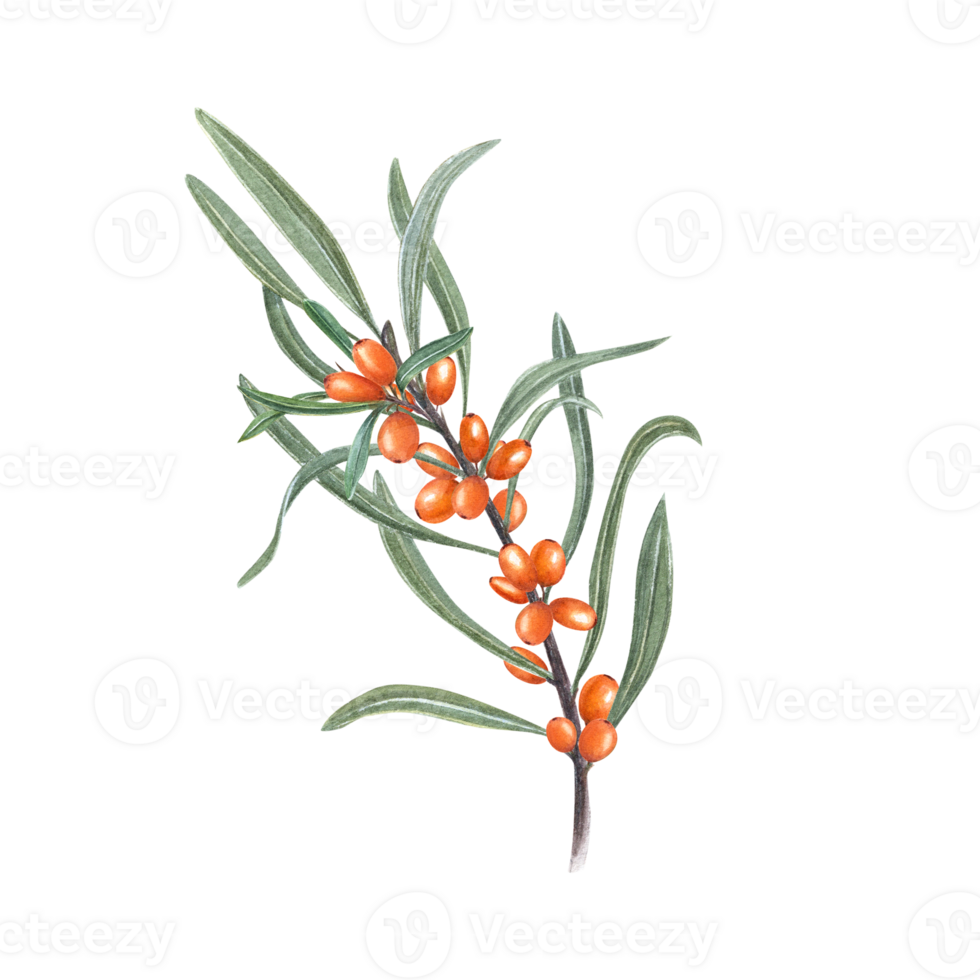This detailed illustration appears to be of a plant featuring thin, elongated green leaves and numerous small reddish-orange buds or berry-like structures. The plant itself is depicted with a central stem from which all the leaves and berries branch off. There are approximately 20 leaves in total, each long and skinny, and a similar number of reddish-orange buds resembling the size and shape of black beans, but with a distinct glossy appearance highlighted by white specular reflections. At each tip of these buds, there is a prominent black dot. The overall shape of the plant is vertical, with a gentle curve sweeping towards the upper left corner. The illustration has a detailed, realistic style that hints at it being digitally drawn or painted, on a clean white background. Faintly visible in the background is the watermark "VECTEEZY," repeated multiple times. This adds a subtle layer to the image, hinting at its digital origin.